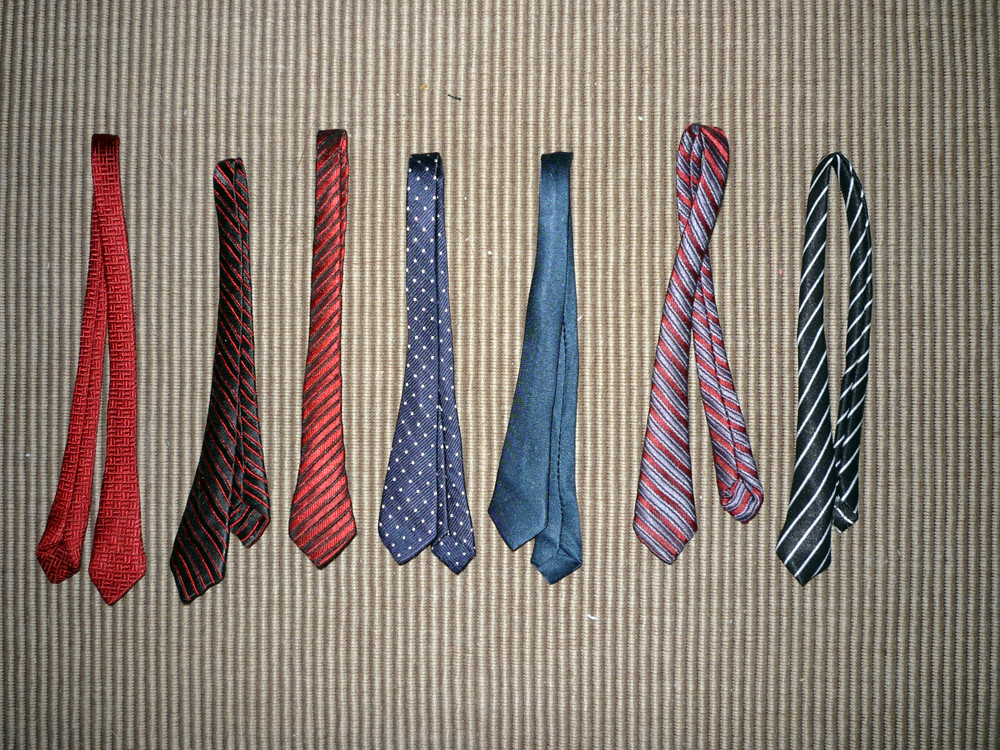This photograph captures a collection of seven ties meticulously lined up on a striped carpet. The carpet, which features a pattern of white and brown stripes, appears somewhat dirty with small pieces of trash and dust scattered across its surface. The photo, taken with a flash, highlights the slightly worn condition of the ties, all of which are relatively thin. From left to right, the ties display a range of colors and patterns: the first is solid red, the second is black with red stripes, the third is red with black stripes, the fourth is dark blue with white polka dots, the fifth is solid blue, the sixth showcases a variation of red and gray stripes, and the final tie is black with white stripes.